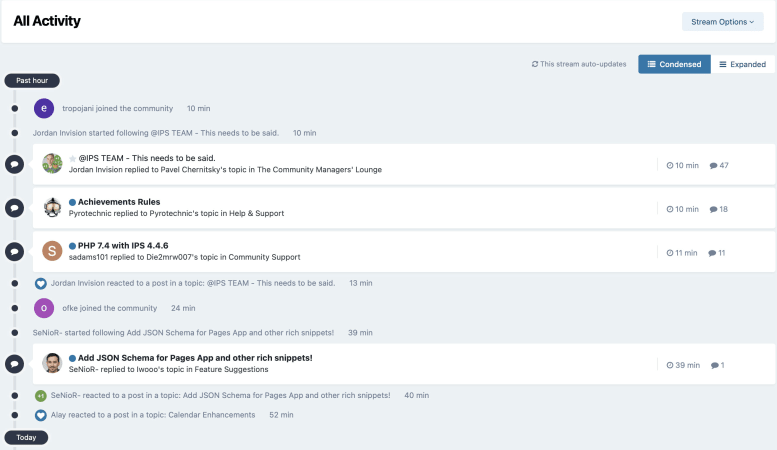This image appears to be a screenshot of a desktop or tablet interface showcasing a community message board. In the upper left-hand corner, there's a label that reads "All Activity," indicating that the feed displays a complete list of user actions or messages. On the upper right-hand corner, there's an option labeled "Stream Options" with a downward arrow, suggesting a dropdown menu for additional settings or filters.

The message board itself seems to be part of an online community, though the specific type of community is not specified. The background of the interface is a very light blue, which contrasts with the individual message cards that have white backgrounds. To the left side of the image, there is a timetable feature. At the top of this timeline, it says "Past hour," and it continues to list entries chronologically down to the bottom left-hand corner, which reads "Today." This timetable allows users to see the comments or activities arranged in temporal order, providing a clear view of the community's ongoing discussions and interactions.